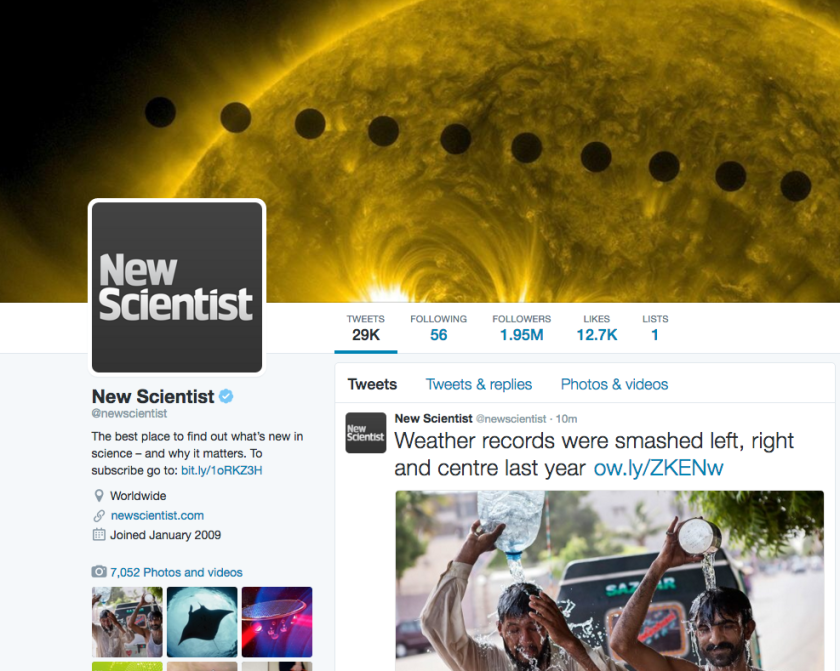This image showcases the official TwitterX page of New Scientist, a science journal. At the top of the screen, there's a visually striking banner featuring a planet illuminated by a yellow glow against a black background, with a diagonal line of black polka dots crossing through the image. In the center of this banner is a dark gray square outlined in white, containing "New Scientist" in bold white text.

Below this banner, the page includes navigation options labeled: Tweets, Following, Followers, Likes, and Lists, each accompanied by corresponding numbers. Beneath these options is a prominent article entitled "Weather Records Were Smashed Left, Right, and Center Last Year." The article is accompanied by an image of two men drenched with bottled water on a sunny afternoon, with a street scene in the background. 

Above this article preview are further navigation options: Tweets, Tweets & Replies, and Photos & Videos. On the left side of the screen, next to the blue verified checkmark, it says "New Scientist" followed by the tagline "the best place to find out what's new in science and why it matters." Additionally, there's a hyperlink inviting users to subscribe for more content.